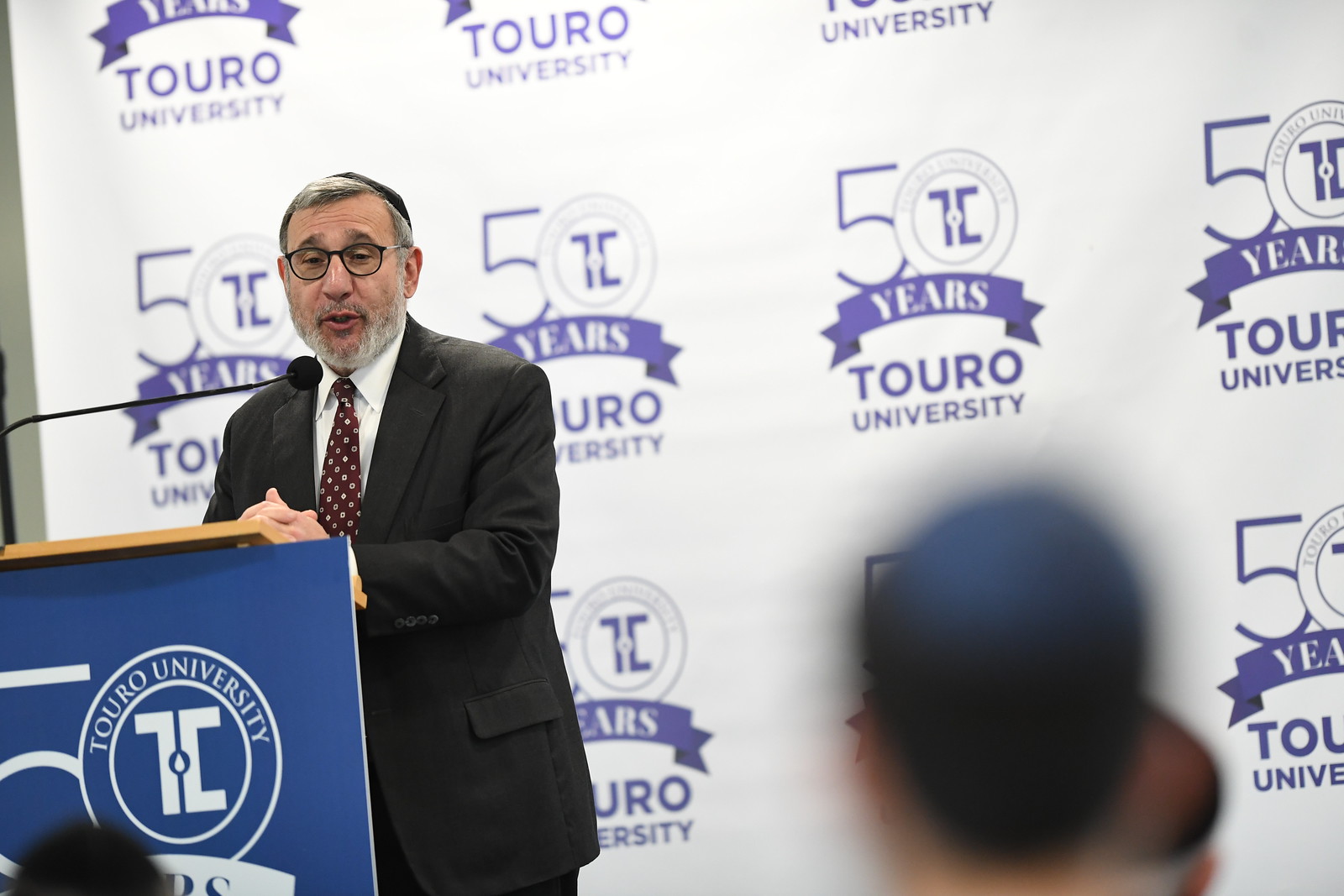The image depicts an older man, distinguished by his graying hair, beard, mustache, and glasses, standing at a blue lectern with a microphone. He is wearing a yarmulke, a dark suit jacket, a white shirt, and a red and white tie. The lectern displays a logo consisting of a blue "50" beside a circle with "years" written in white, and "Touro University" in blue. This logo is also prominently featured on a white backdrop behind him, repeated in purple, indicating a celebratory event such as the university's 50th anniversary. The setting appears to be a formal university gathering, perhaps a graduation or a significant assembly, given his prominent speaking role. In the foreground, the heads of attentive audience members are faintly visible.